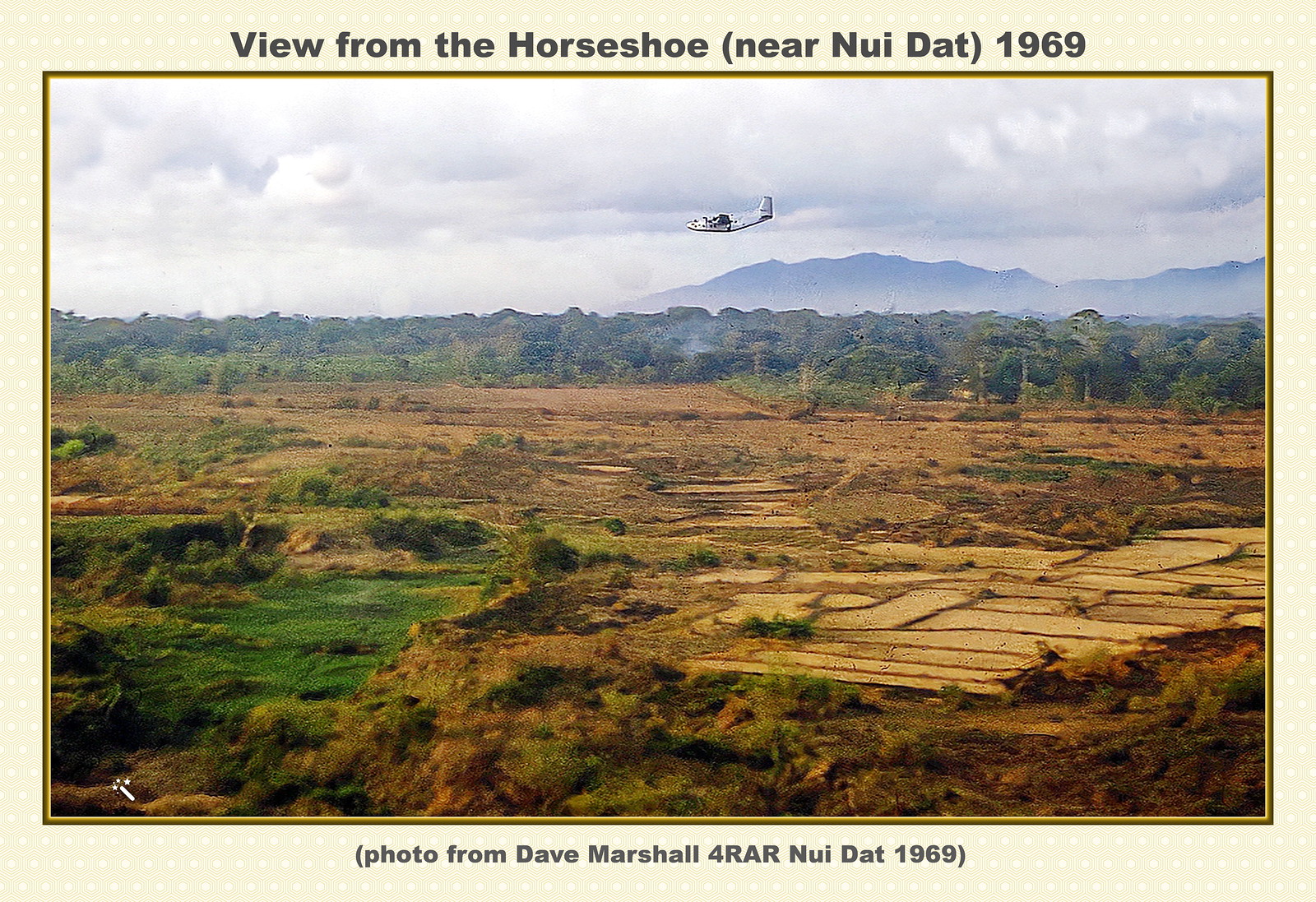This photograph showcases a white airplane, possibly thick-bodied for airdrops, flying horizontally to the left over a vast field. The foreground of the image reveals the ground below, characterized by a mix of green and brown grass, patches of green plants, and extensive areas of brown soil. In the lower-right section, there are farming plots bordered by stone and dirt, currently devoid of vegetation. Beyond the main field, a line of trees stands in the mid-ground, giving way to hills in the distant background. The sky is dense with white and dark clouds. The photograph is framed with a light brown border, featuring black text that provides context. At the top, it reads "View from the Horseshoe, near Nui Dat, 1969," while the bottom text states, "Photo from Dave Marshall for RAR, Nui Dat, 1969." The overall scene, likely from the Vietnam era, captures the expansive and open landscape beneath the flying aircraft along with a hint of smoke in the image.